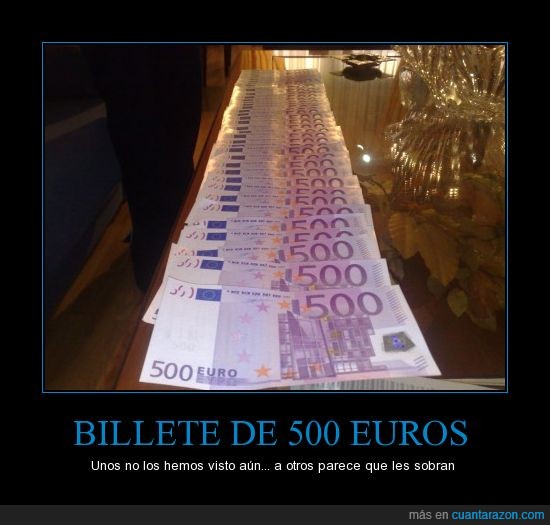In this poster, featuring a black background with a thin blue outline around the central image, an intricate display of 500 Euro banknotes is shown. The main image showcases a long, seemingly endless row of these bills, which are elegantly spread out from the center, creating a cascading effect that reaches towards the top of the image. The 500 Euro notes prominently display the number "500" in bright purple along with stars encased in a circular design, in shades of purple and orange. These bills rest on a reflective surface suggestive of a glass table, adding a touch of sophistication to the scene. The black border surrounding the image contains white text, including "Billet de 500 Euros" in blue capital letters, indicating this poster might be in French or Spanish. At the bottom right, the URL "cuantarazon.com" in smaller print suggests a promotional or informational context, potentially an advertisement where one could win a large sum of money.